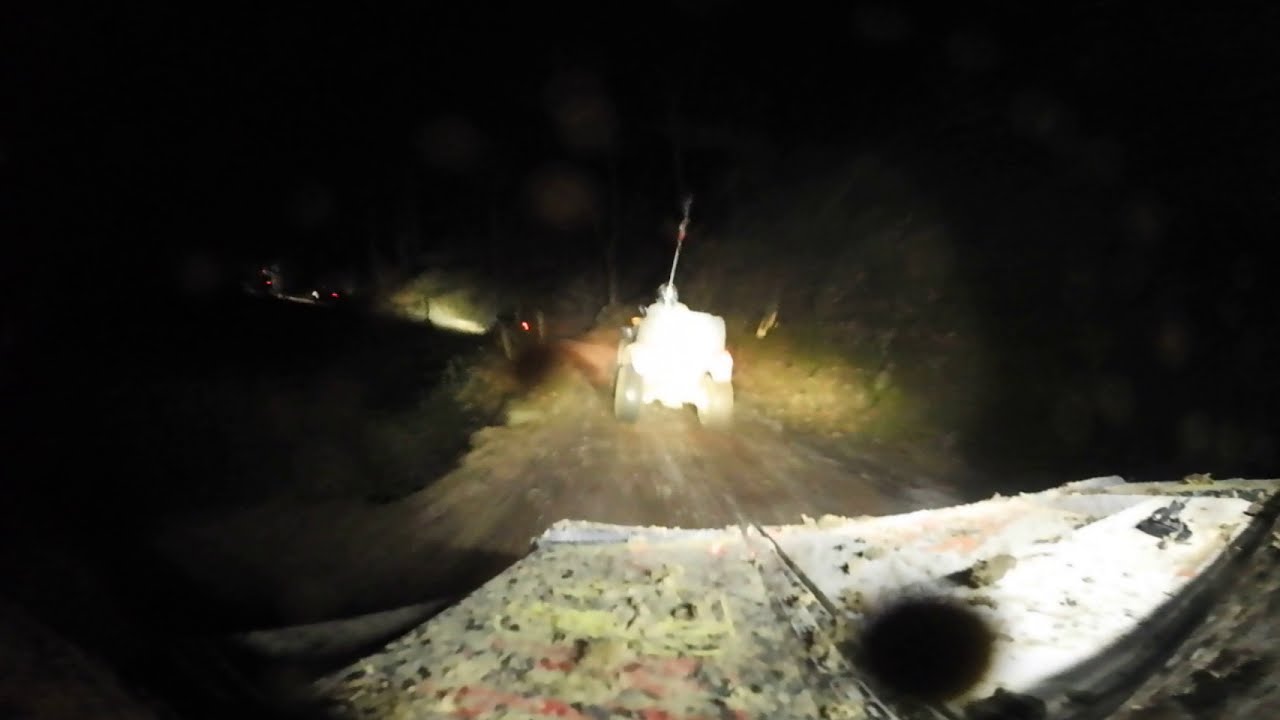In the middle of a dim, muddy dirt road at night, an off-road, military-style vehicle with large, wide back tires navigates the slick terrain. The vehicle, illuminated by a bright light in the rear, exposes a distinct antenna with an oddly shaped object at its top. Its blocky silhouette is whited out due to the intense beams from the headlights of another vehicle behind it, casting pools of orange and yellow light on the muddy ground ahead. The tires reveal contrasting colors; the left tire appears black, while the right one, muddied from the journey, adopts a brownish hue. Surrounding this vehicle are patches of black, with an assortment of yellow, pink, black, and white blotches visible on a painted surface near the lower right corner. Along the winding road, several more vehicles can be discerned by their red taillights and bright headlights cutting through the darkness. The scene is enveloped in an overwhelming blackness, especially in the upper corners and the left side of the photo, highlighting the nighttime setting. The faint presence of trees outlines the sides of the road, adding to the rugged, outdoor environment. Despite the image's blur and abstract elements, it captures the essence of a nocturnal, off-road adventure.